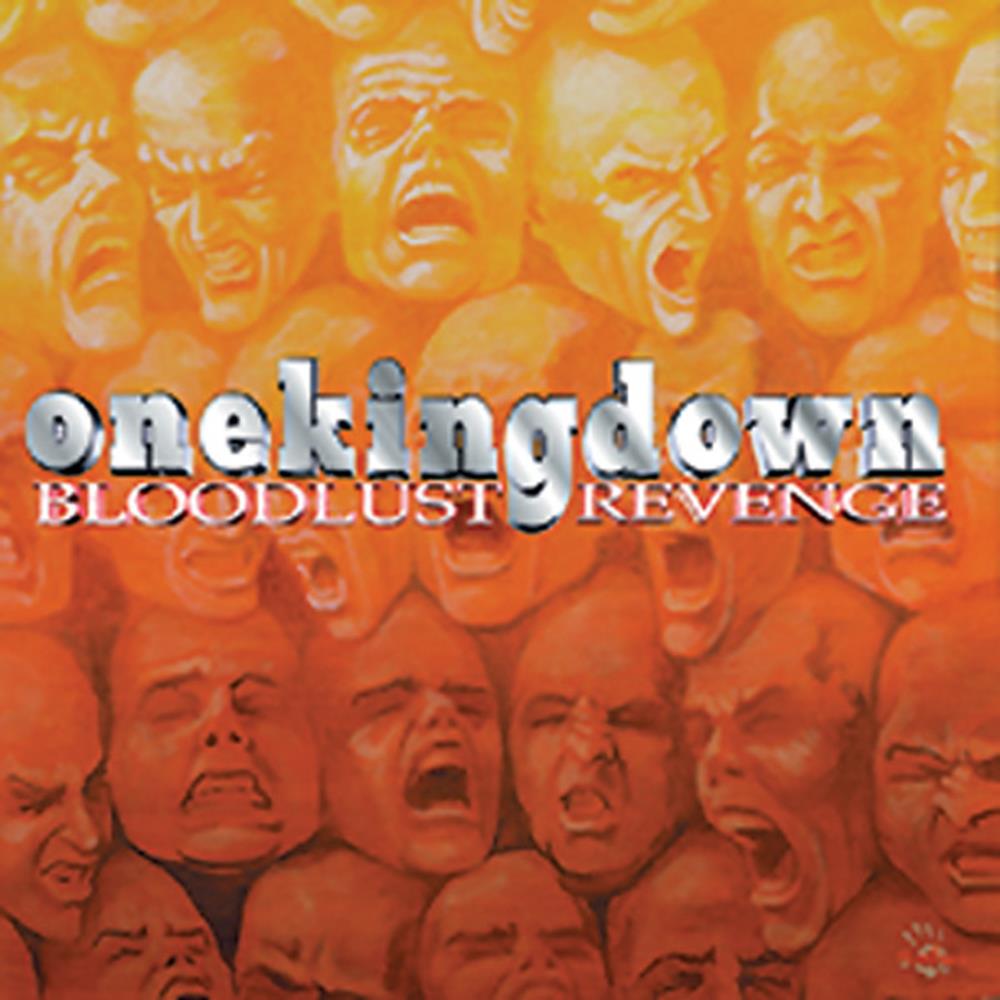This image, likely an advertisement or album cover, is a square composition featuring a gradient background transitioning from light yellow at the top to deep red at the bottom. The backdrop is densely packed with rows of men's heads depicted in extreme anguish, their mouths open and eyes shut, giving a sense of pain and torment. The heads, arranged in about four or five rows with approximately five or six heads per row, are slightly varied in orientation but uniformly convey a scream or yell. The background's orange-reddish hue grows darker as it descends, enhancing the intensity of the depicted agony.

Centrally positioned on this harrowing scene is a prominent piece of silver text. The main line reads "One King Down" in a larger, silver block font, lacking spaces between the words. Below this, in a smaller font and all capitals, it reads "Bloodlust Revenge," with a distinctive lowercase 'G' in "Bloodlust" that descends, separating the word from "Revenge." The composition is completed with a small white handprint insignia in the lower right-hand corner, adding a final striking element to the image.